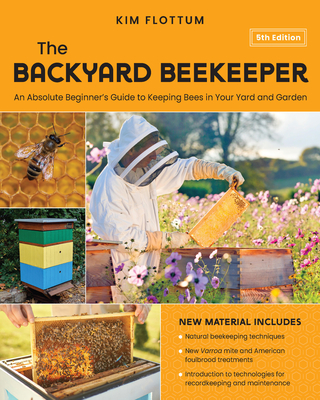This is the cover of "The Backyard Beekeeper, 5th Edition: An Absolute Beginner's Guide to Keeping Bees in Your Yard and Garden" by Kim Flottam. The cover is divided into several sections with a predominantly golden-yellow background. At the top, a full-width yellow rectangle prominently features the author's name, Kim Flottam, in black text. Below this, in white text, it states "5th Edition," followed by the book's title in black.

The bottom part of the cover is divided into several images and a text box. On the left side, there are two square photographs. The top square displays a close-up of a bee with its wings extended, standing on a honeycomb. Directly below this, another square features a beehive with multiple color-coded sections—bright blue at the bottom, then light yellow, dark green, and brown at the top—all set against a background of greenery.

To the right of these images is a larger square photograph of a beekeeper in full protective gear, including netting, holding a piece of honeycomb. This beekeeper stands in front of bee boxes amidst a field of pink flowers. In the lower-left corner, there's a smaller image of a hand (without a glove) lifting a honeycomb panel out of a hive filled with bees.

In the bottom-right corner, a golden-yellow rectangle lists the new materials included in this edition: Natural Beekeeping Techniques, New Varroa Mite and American Foulbrood Treatments, and an Introduction to Technologies for Recordkeeping and Maintenance.